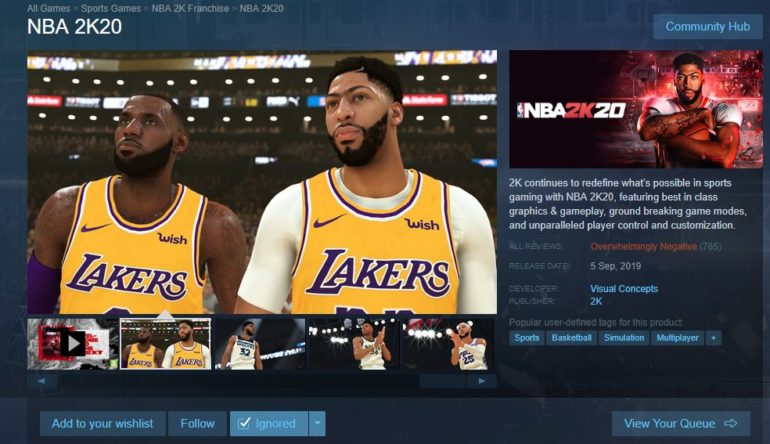A screenshot from the Steam platform displays the listing page for the game NBA 2K20. The interface features a blue background at the top, housing navigation options in light gray text, including "All Games," "Sports Games," and specific franchises like "NBA 2K." In focus is NBA 2K20, highlighted with several screenshots, prominently showing two players from the Los Angeles Lakers team.

Below the main screenshot, there are additional thumbnails for toggling through more images of the game. Interactive buttons allow users to add the game to their wishlist, follow it, or ignore it—the latter currently checkmarked. In the bottom-right corner, an option labeled "View Your Queue" with a rightward arrow is visible.

To the right of the main image, the game title "NBA 2K20" appears alongside another image of a basketball player holding a ball. Beneath this image, a description reads: "2K continues to redefine what's possible in sports gaming with NBA 2K20, featuring best-in-class graphics and gameplay, groundbreaking game modes, and unparalleled player control and customization."

The game has garnered "Overwhelmingly Negative" reviews from 765 users. Further details include a release date of September 5, 2019, with Visual Concepts as the developer and 2K as the publisher. Popular user-defined tags for NBA 2K20 include sports, basketball, simulation, and multiplayer.